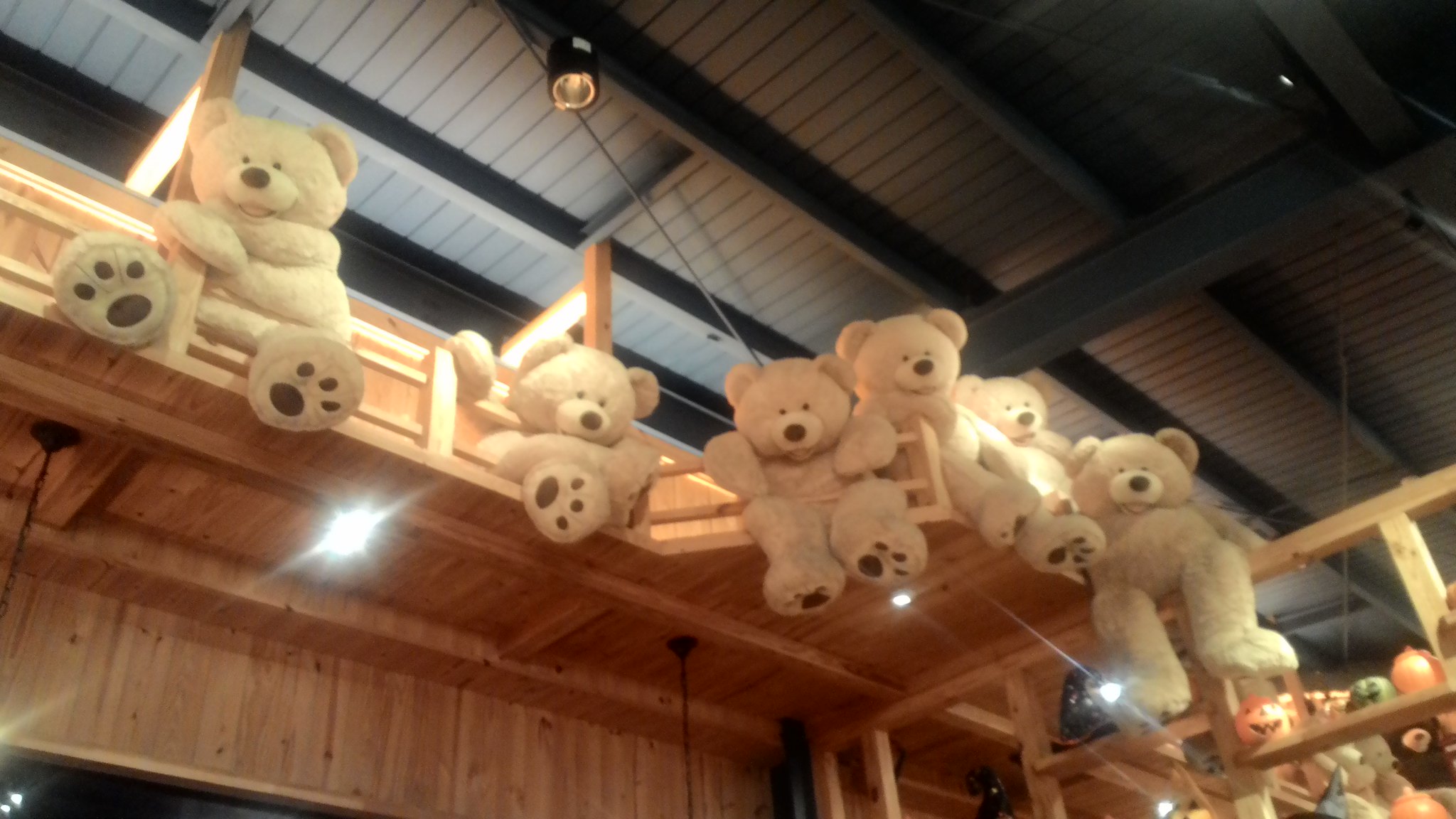This photograph captures an upward view of the interior of what appears to be a toy store. The ceiling features black-painted, exposed wood beams. Prominently displayed on a wooden structure resembling a catwalk or balcony, a row of six identical, off-white teddy bears with dark brown noses, eyes, and paw prints on their feet can be seen. They are positioned along a wooden fence that runs across the top of the structure, with some bears hanging by their feet and others appearing to hug the railing or peek between the fence slats. These cheerful bears seem to be observing the scene below, adding a whimsical touch to the store's decor.